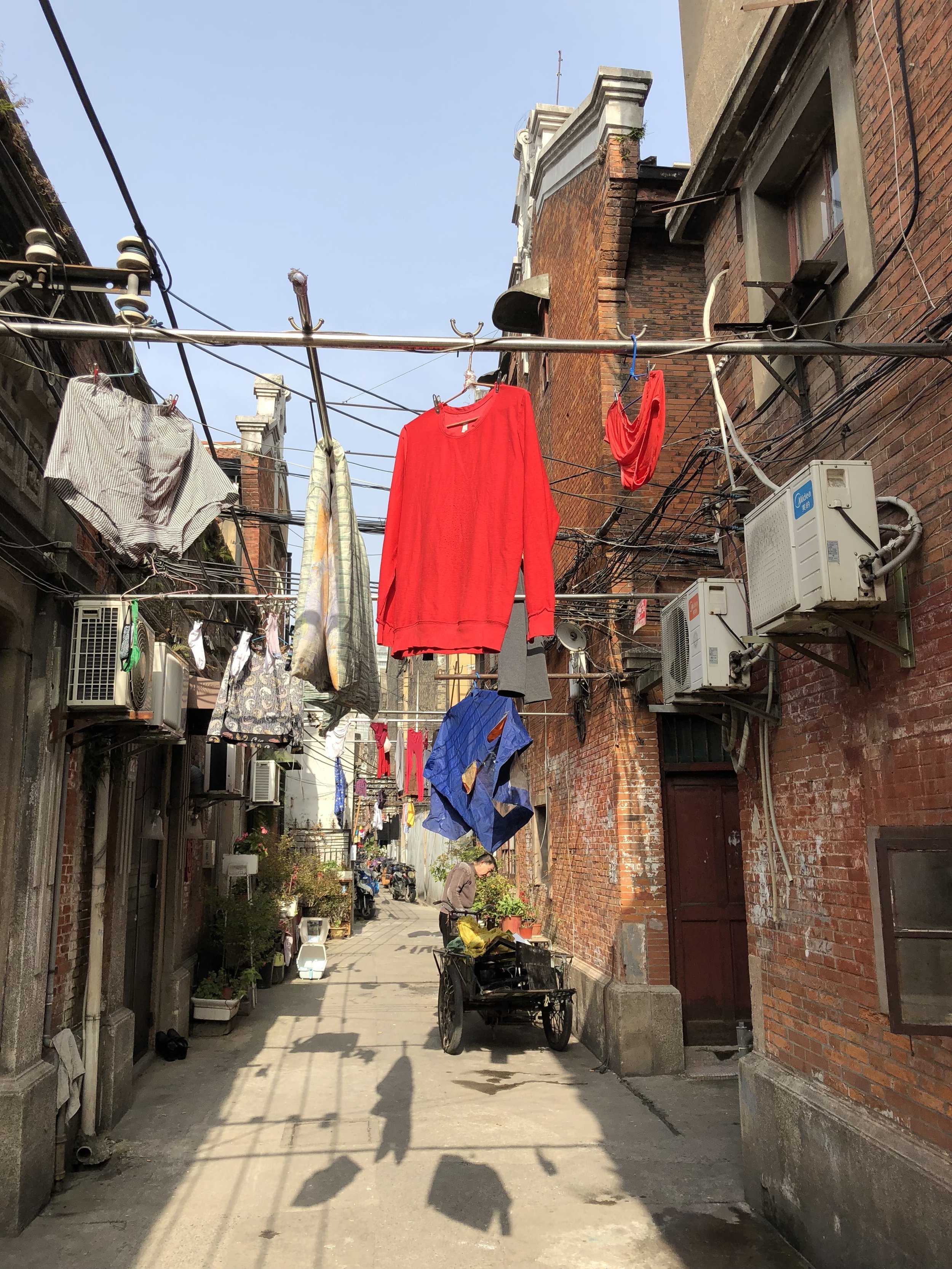The image depicts a dingy alleyway framed by run-down, poorly maintained brick buildings on both sides. The clear, light blue sky above is free of clouds, providing a stark contrast to the cluttered scene below. The buildings are adorned with numerous silver pipes and air conditioning units, some of which have red, blue, and green labels. The front of the buildings features red bricks accented with gray cement around the windows.

On the right side, there's a brown door, next to which a black carriage filled with assorted green and yellow items can be seen. The ground is a gray concrete pavement, slightly dirty and littered with miscellaneous items.

Clothing hangs prominently from metal poles that stretch between the buildings. A red shirt on a pink hanger, a pair of red underwear or similar item on a blue hanger, a blue shirt, and multiple pairs of red pants are visible. There is also a pair of tan boxers and two tan and white shirts. Two white doves perch on the laundry setup. Additionally, plants—mostly green—are scattered on the left side, enhancing the sense of a residential area.